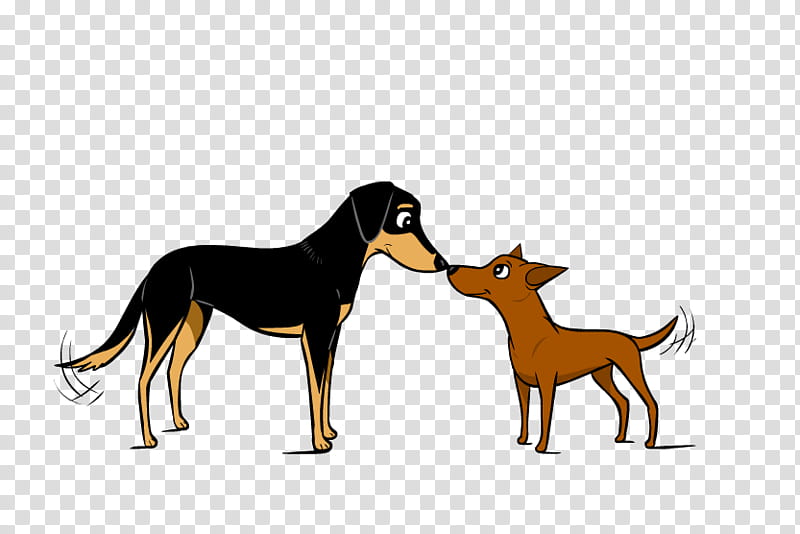This image is a detailed graphic illustration featuring two stylized dogs set against an intricate, repeating checkerboard background of small gray and white squares. On the left is a black and tan Dachshund-like dog, with bright, expressive eyes and a smiling expression. Its body and tail are primarily black, with brown accents around the muzzle, under the tail, and on the lower parts of its legs. The dog seems to be wagging its tail happily. Facing this dog on the right is another dog, slightly taller and brown in color, also with a happy demeanor. This second dog is simpler in appearance, with perked-up ears and a matching gaze as it touches noses with the black and tan dog. The entire backdrop is an op-art checkerboard pattern that stretches across the image, enhancing the engaging and playful interaction between the two dogs.